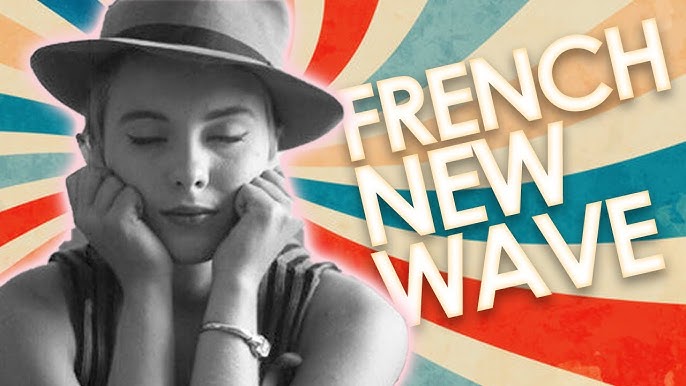The image presents a close-up black and white photograph of a young woman, depicting her from the shoulders up with a vintage, artistic flair. She is wearing a brimmed cowboy-style hat, accentuating her closed eyes and chic winged eyeliner. Her expression is gently contemplative, with both fists resting adorably on her cheeks. A lit cigarette adds a touch of classic rebellion to her pose. The background features a striking spiral pattern with alternating stripes of white, red, blue, cream, and yellow, all converging around her. On her right wrist, she sports a bracelet. Dominating the right side of the image is the text "FRENCH NEW WAVE" in large, bold letters—white with a gradient transitioning to orange on the edges. This captivating blend of elements creates a striking homage to the iconic French New Wave style.